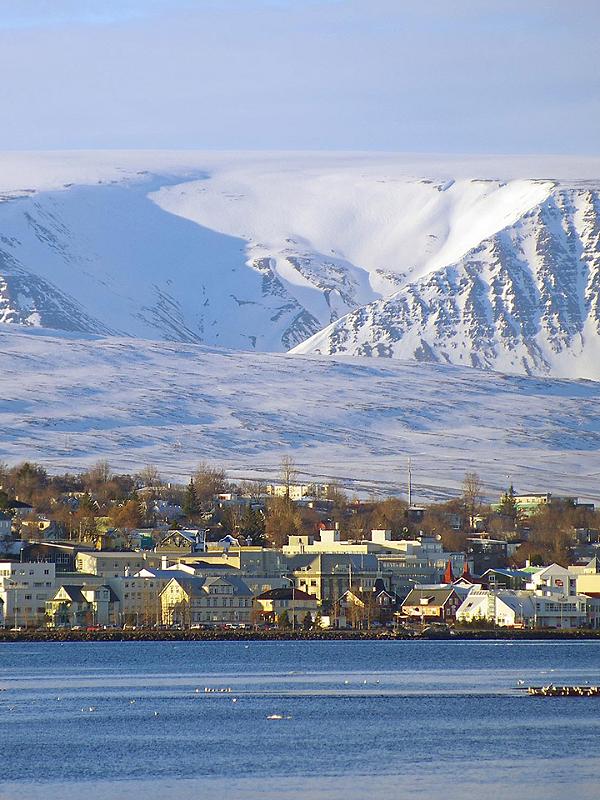This is a color photograph in portrait orientation, capturing a detailed and picturesque shoreline scene of Akureyri, Iceland. In the foreground, a medium blue ocean stretches across the bottom quarter of the image, dotted with white birds, likely seagulls, some resting on a brown outcropping of land near the right side. Just above the water line, a bustling townscape fills the midsection of the frame. 

The town features a mix of two to three-story wooden structures with angled roofs, some painted yellow, and several modern three to four-story buildings. Commercial buildings also punctuate the skyline, with a two-story structure standing out on the right. A line of cars is parked against a fence along the shoreline, indicating a busy coastal community. Intermittent goldish-brown trees add a touch of autumn color to the scenery.

Behind the town, the landscape ascends to a snow-covered hillside, contributing to the wintry atmosphere. This is further accentuated by a towering mountain range with dark gray peaks and snow-laden valleys, which occupies the upper portion of the photograph, reaching into a clear, light blue sky. The photograph embodies a sense of realism, capturing the serene yet lively essence of a coastal town set against a dramatic, mountainous backdrop.